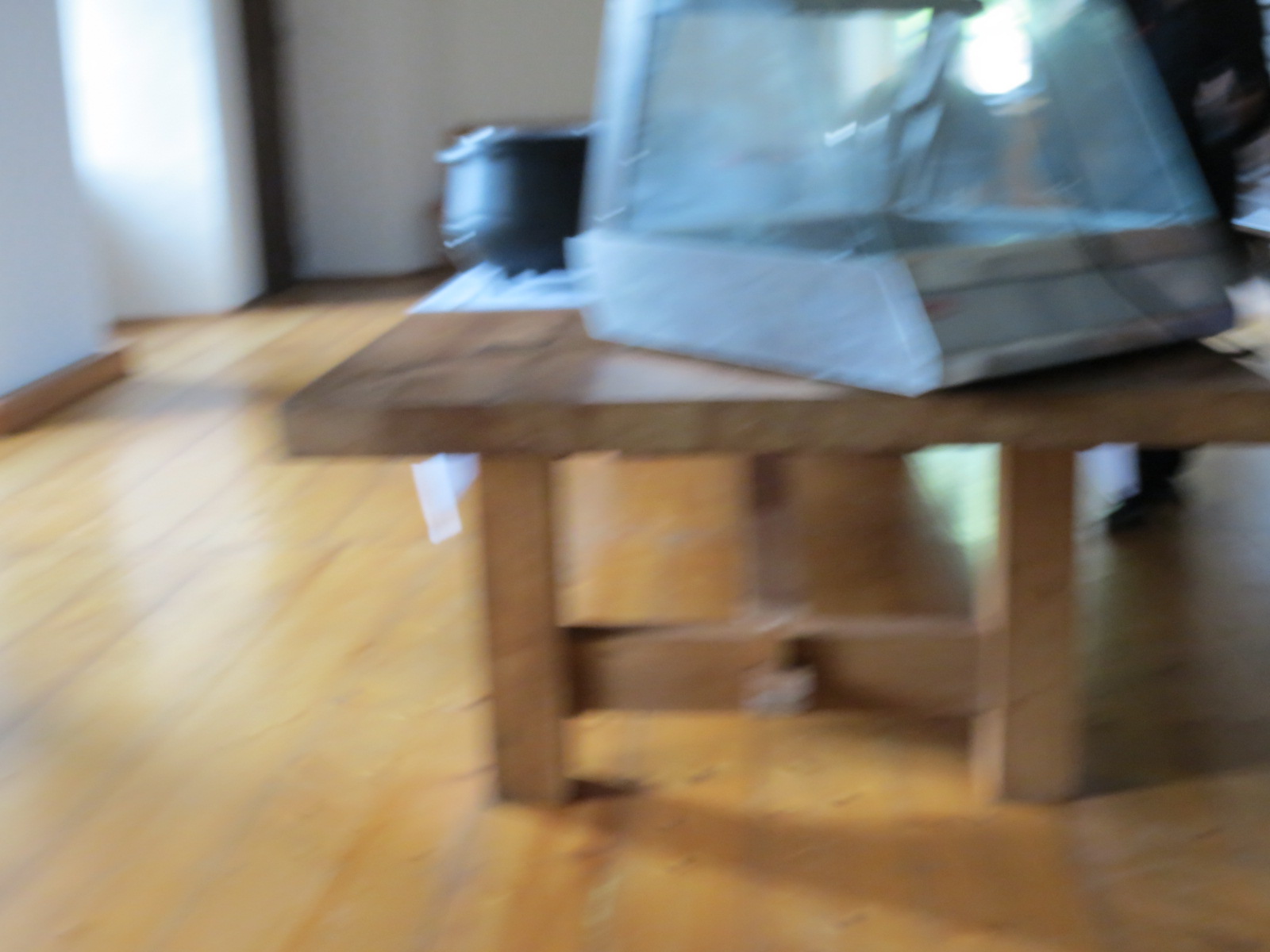This very blurry photograph depicts an indoor scene featuring a table set on a light honey-colored wood floor with dark lines demarcating each tile. The floor's hue closely matches the table, which is of solid but shoddy construction, slightly darker than the flooring. White walls are visible in the upper left corner, accompanied by matching baseboards. On the table, which occupies a central position in the mostly empty room, there is a large, indistinct item with a silver base and a glass or translucent enclosure, possibly resembling a piece of chemical equipment or an incubator. This object includes a control panel, with a red button situated on the upper left-hand side of the panel. To the table’s upper right, a blurry black cauldron-like pot can be seen, adding an element of curiosity. Additionally, the outline of a person dressed in dark clothes is vaguely visible at the back right edge of the table, though the blurriness conceals their actions.